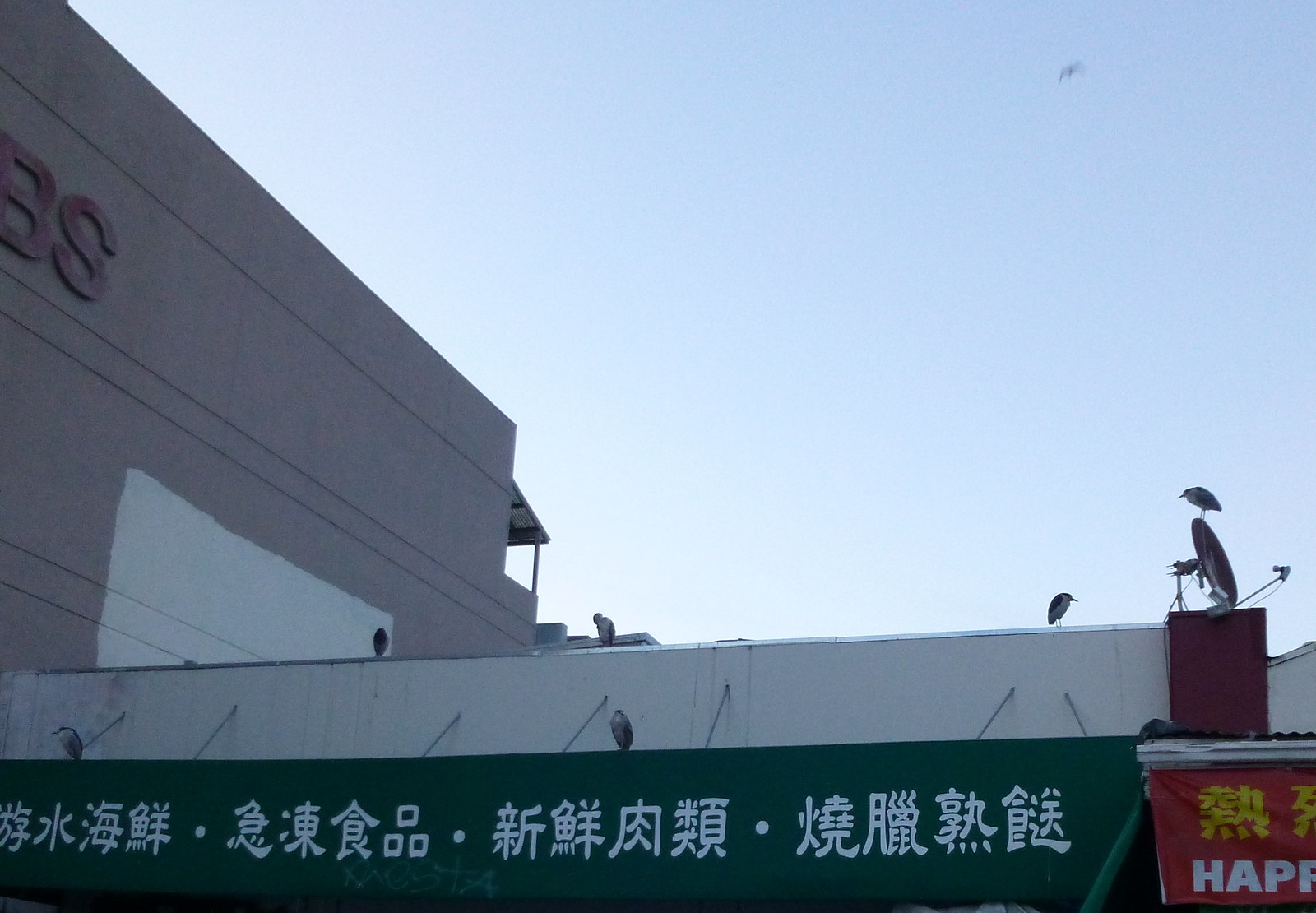This photograph captures an outdoor scene featuring multiple buildings in a foreign country, dominated by a prominently basic white building angled down towards the center of the picture. On the top left corner of this building, the letters "B" and "S" can be seen, suggesting they are part of a larger, unfinished word, and the structure notably lacks windows or doors on the visible side. In the foreground, a green banner with Chinese characters extends horizontally across the lower part of the image, partially obscured by what appears to be a wall or barrier. To the right, a red-colored sign with white English letters "H-A-P," seemingly part of the word "happy," accompanies a podium or box with a small satellite dish on top, also featuring more Chinese characters in gold. The scene is enriched by several birds perched on the various roofs and on the satellite dish, under a clear, light blue sky.